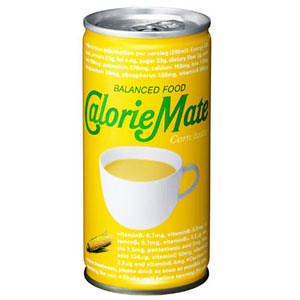The image presents a meticulously designed 3D rendering of a drink can set against a pure white background, emphasizing the can as the focal point. The can features a standard cylindrical shape with a classic silver rim at both the top and base, which subtly protrude outward. The top of the can is adorned with a silver pop tab, adding a touch of realism to the rendering.

The body of the can is strikingly bright yellow, accompanied by white text at both the top and the bottom, though the latter is partially obscured and unreadable. The upper section, however, remains clear, hinting at the product's branding. Prominently displayed on the can’s surface is a detailed illustration of a white teacup filled with a pale yellow liquid, suggesting a soothing beverage. Adjacent to this image, in the bottom-left quadrant of the can’s design, an ear of yellow corn is vividly illustrated, complete with verdant green husks, symbolizing wholesome, natural ingredients.

Adding to the narrative, green text declaring "Balanced Food" and "Calorie Mate" enhances the can's lower section, conveying the drink's nutritional and brand identity.